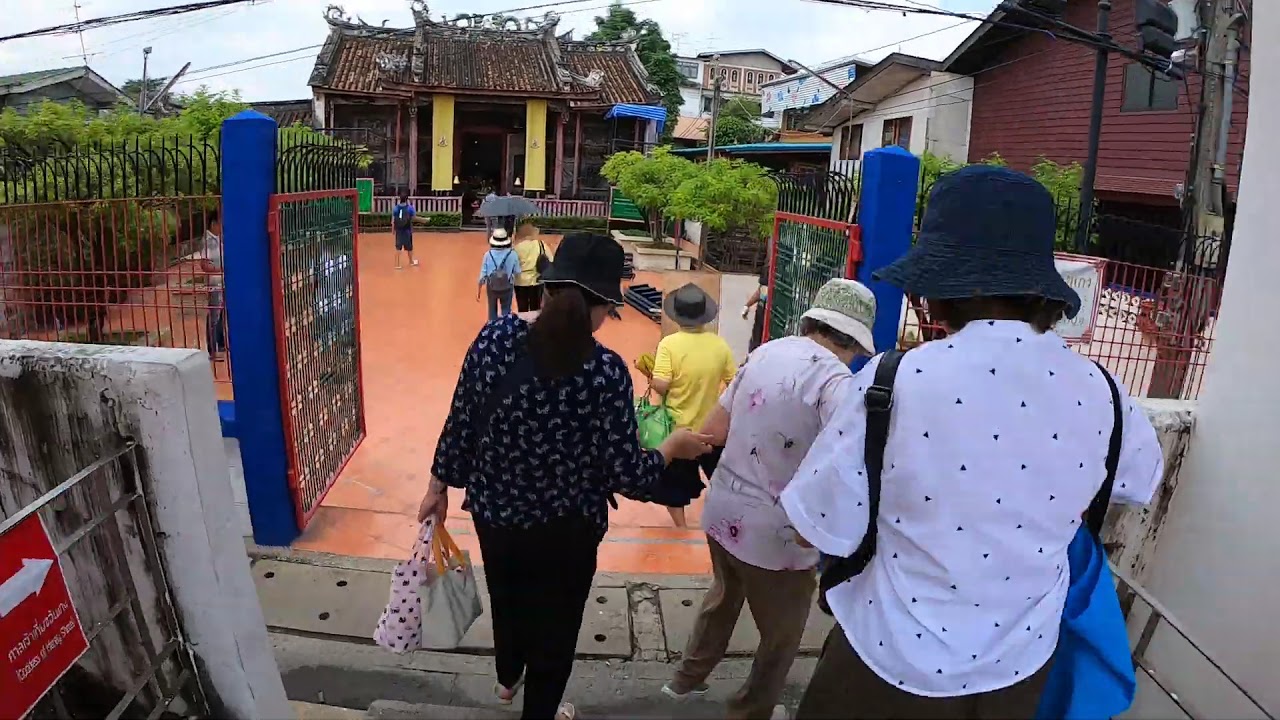This horizontally aligned rectangular image captures a bustling scene of tourists disembarking from a platform in what appears to be an Asian village, likely a tourist site. The central focus is on three women in the foreground, stepping off a gray concrete area that resembles the base of a set of steps and onto a glossy orange tiled path. The woman on the right wears a blue bucket hat and a white patterned shirt, while another woman with a black bucket hat, dark ponytail, blue and white patterned shirt, and black slacks assists an elderly woman dressed in a short-sleeve white patterned shirt and brown pants. They are passing through distinctive black metal gates with a cut-out design and red borders, connected to blue posts embedded in the ground.

The environment around them features additional details, such as buildings to the right and ahead, including a notable house of worship with yellow tapestries and traditional Asian designs. The sky appears partly sunny with a mixture of blue and clouds, although the overall atmosphere suggests it could be a cloudy or rainy day, given the presence of people with umbrellas. A red sign with a white arrow directs the flow of tourists towards a prominent building in the background, which has a brown roof and a yellow facade, further emphasizing the culturally rich and peaceful ambiance of the scene.